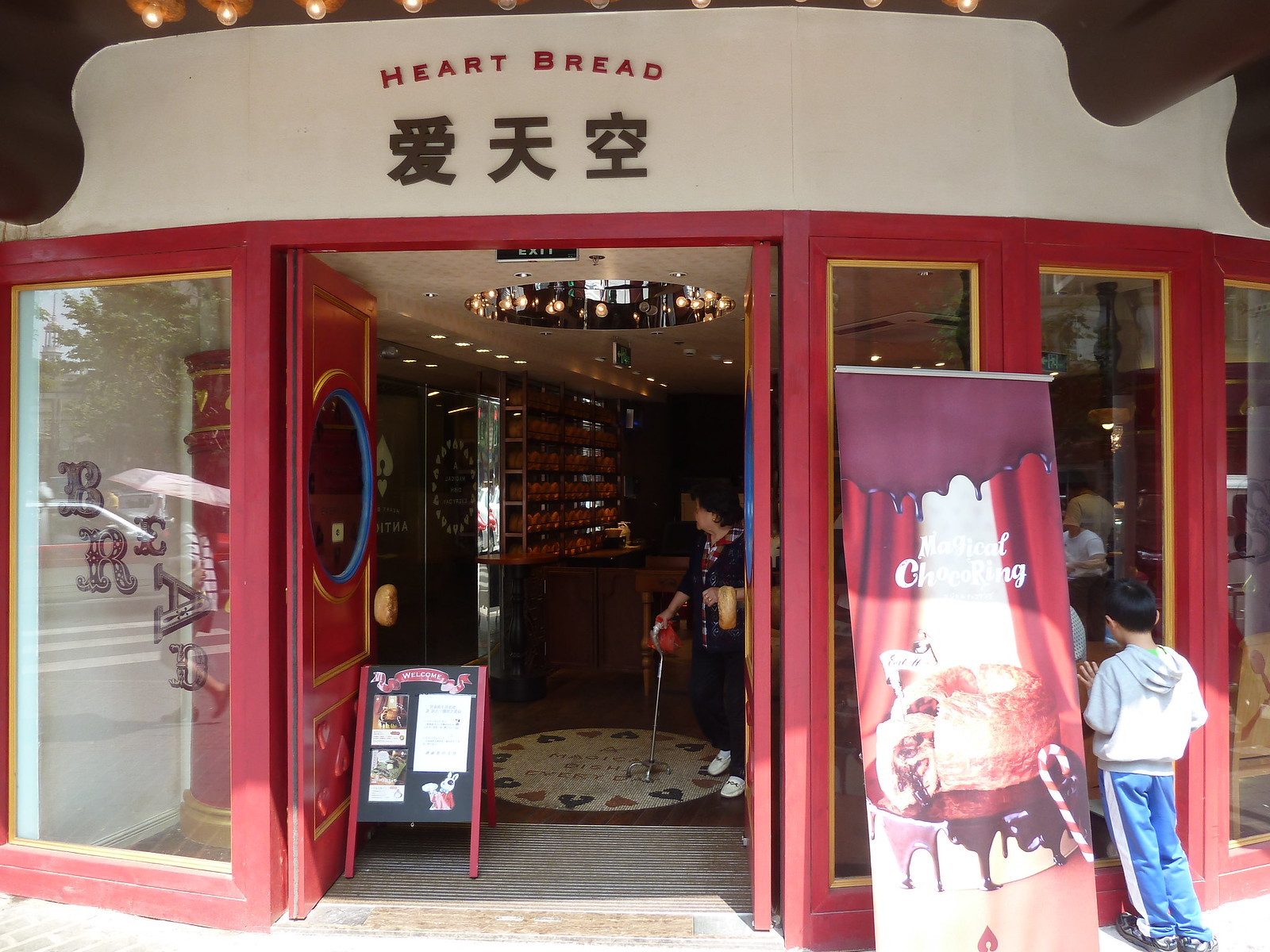This image captures the vibrant storefront of a red and white Asian bakery named "Heart Bread," highlighted by signage in both English and Japanese kanji characters. The bakery features large windows framed in red, enhancing its inviting allure. Two pink-framed double doors at the entrance are propped open, welcoming visitors inside. Just outside, a sandwich board sign with various papers and the phrase "Magical Choco Ring" showcases the day's specials. To the right of this sign, a young boy dressed in a sweatshirt and blue pants leans against the window, gazing intently at the bakery's delicious offerings. Inside the open doors, a lady wearing white sneakers and a black outfit, aided by a cane, explores the bakery. The scene also includes a round floor decal with whimsical drawings and a glimpse of the pastry display to the left. The lively atmosphere is accentuated with playful lettering spelling "BREAD" in a scattered fashion on the left window. Overall, the bakery's colorful exterior and the bustle of activity hint at the delightful treats within.